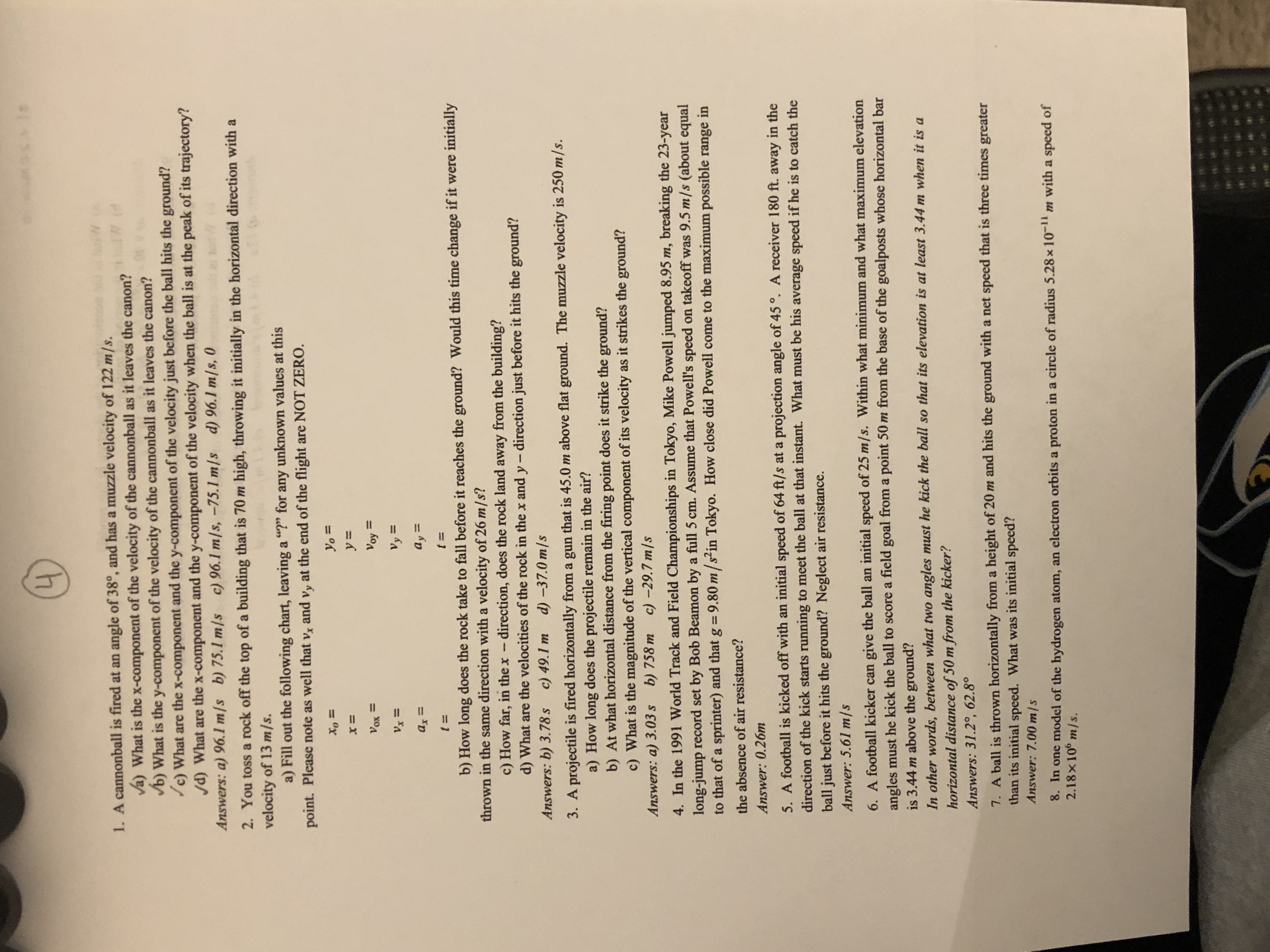The image is a photograph of a math or physics homework page, turned sideways, making it difficult to read. It consists of dense black text on a white sheet, featuring a total of eight questions, many of which are divided into multiple sub-parts. The questions revolve around projectile motion and velocity calculations, covering scenarios like cannonballs being fired at a specific angle, rocks thrown from a building, and footballs kicked at particular speeds. For example, one question discusses a cannonball fired at a 38-degree angle with a muzzle velocity of 122 m/s, asking for the x and y components of its velocity at various points in its trajectory. The answers to these questions are provided directly below each query. Additionally, there's a penciled-in and circled number four at the top of the page, indicating it might be part of a test or a homework set.